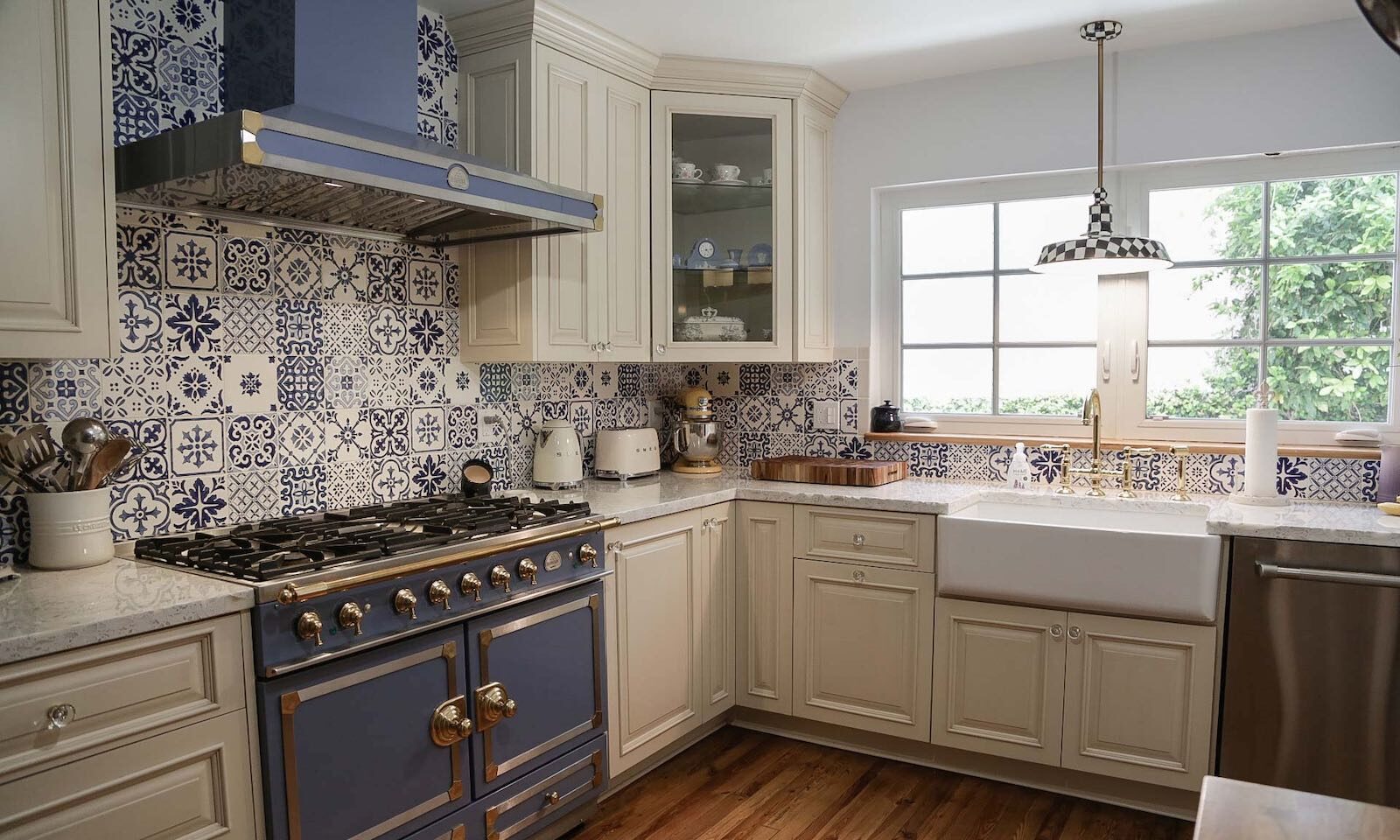The image captures the interior of a beautifully designed and well-maintained kitchen, bathed in natural light streaming through a large window on the right-hand side, which offers a view of ivy and a tree in the backyard. The kitchen features cream-colored cabinets accented by tan wood and a set of granite countertops. A prominent element is the unique Wedgwood blue stove, adorned with silver and brass metallic accents, which sits below a high-end blue ventilation system with integrated recessed lighting.

Above a white marble double sink hangs an eye-catching black and white checkered lamp, its wiring encased in a green and gold tube, casting light over the sink area. The ornate backsplash is composed of various 3x3 tiles, each displaying different intricate blue and white patterns, including floral and geometric designs.

The kitchen is neatly organized, furnished with common household appliances such as a toaster, coffee pot, kettle, food mixer, paper towel dispenser, and a dishwasher. A container filled with ladles, spatulas, and other utensils sits on the countertop, next to a cutting board. The countertops also host a vase with numerous ladles and spatulas, adding a practical yet decorative touch.

Hanging from the wall, you'll find both closed cream-colored cabinets and a singular glass-front cabinet displaying tea sets, a clock, and other decorative items. The gold fixtures and handles add a touch of elegance, completing the sophisticated yet cozy ambiance of this kitchen.